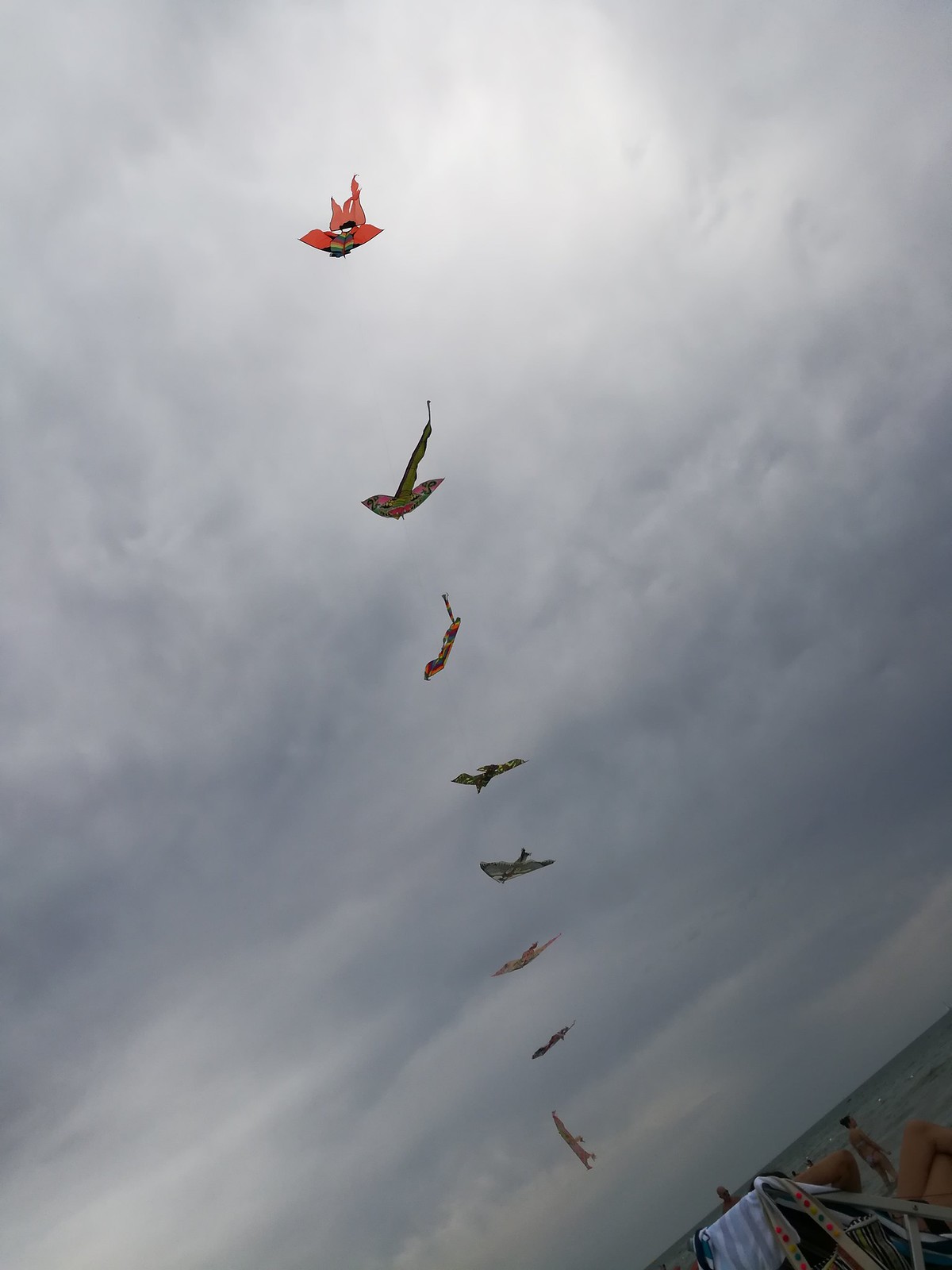This image captures a cloudy, overcast day at what appears to be a beach or lakeside, with the sky taking up about 90% of the frame. The photograph is taken from the ground at a tilted, portrait angle, focusing upwards into a dull, gray sky dense with clouds, suggesting an impending storm. In the bottom right corner, there is part of a beach chair visible, showing the back and the metal frame of the seating area. A person is sitting in the chair, with crossed legs and an elbow in sight. In front of this person stands another individual, possibly a male with short brown hair, wearing a bathing suit, near the edge of what seems to be dark blue water—the exact nature of the water body is ambiguous, but it is either the ocean or a large lake.

Additionally, an eye-catching array of eight kites fills the sky in a vertical formation. The strings and kite handlers are not visible, likely due to the photo's resolution and angle. The kites are multicolored and varied in design: the topmost kite is reddish-orange, followed by a multicolored one resembling a snake or lizard, and others are in shades of green, red, yellow, and more. Some kites suggest bird-like shapes, while others are abstract and non-specific. The colorful pattern creates a stark contrast against the moody clouds, adding a whimsical touch to the otherwise somber scene.